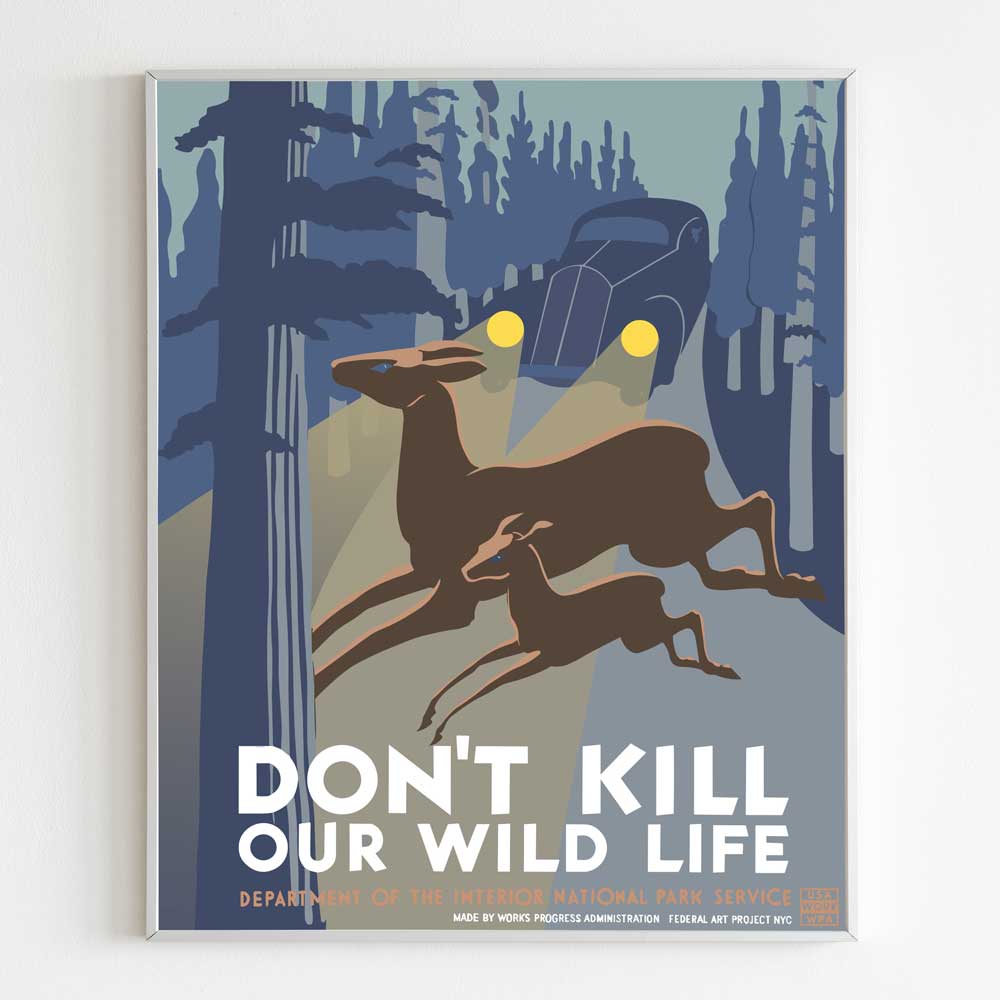The image depicts a framed illustration hanging on a white wall, encased in a matching white frame. The centerpiece of the illustration is a vintage blue car with yellow headlights, traversing a gray road from the background to the foreground. Surrounding the road are trees, artistically rendered in blue. In the foreground, two deer—a mother and her fawn—both adorned with brown coats and blue eyes, are leaping across the street in front of the car. At the bottom of the illustration, a compelling message reads "Don't Kill Our Wildlife" in white lettering. Beneath this message, in brown lettering, the illustration is credited to the "Department of the Interior National Park Service." Further below, in white lettering, the illustration is noted as being "Made by Works Progress Administration, Federal Art Project, NYC."